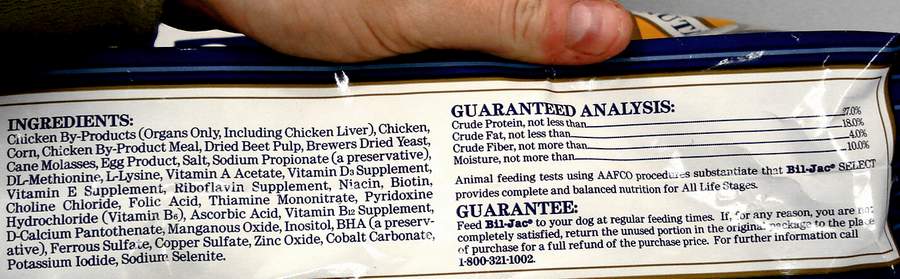Photographic image showing a close-up view of the side of a dog food package. The package features a blue backdrop adorned with a white label bordered with touches of yellow and blue. Prominently displayed on the label are the package's ingredients, which include chicken byproducts, chicken corn, chicken byproduct meal, dried beet pulp, brewer's dried yeast, molasses, egg products, salt, sodium propionate (a preservative), vitamin D, vitamin A, vitamin E, riboflavin, niacin, biotin, choline chloride, folic acid, thiamine hydrochloride, along with crude protein and crude fiber. Also captured in the frame is the thumb of a left hand, indicating someone is holding or adjusting the package.